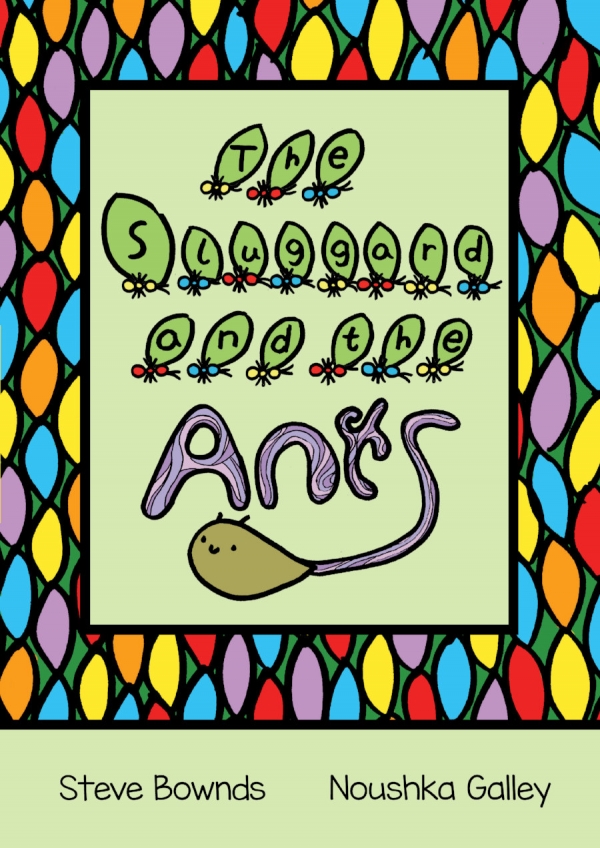The image depicts a vibrant and intricately designed cover of a book titled "The Sluggard and the Ants." The background is reminiscent of a stained glass mosaic, comprising numerous multicolored, almond-shaped pieces in hues of purple, blue, red, yellow, and green, all outlined in black and connected together, creating a crowded yet beautiful tapestry. 

At the center of this ornate design, each letter of the words "The Sluggard and the" is carried by ants of varying colors—red, yellow, and blue—each bearing a leaf. The word "Ants" appears below in large, psychedelic bubble letters in shades of purple with a marbled effect. 

The focus then shifts to a teardrop-shaped creature to the left, presumed to be the "Sluggard," in a dark tan or gray-brown shade, with a smiling face, two eyes, and tiny black antennae. The 'S' in "Ants" cleverly forms the tail of this creature, adding a whimsical touch to the design.

Finally, a light green horizontal strip at the bottom of the cover highlights the names of the author and illustrator in black text: Steve Bounds on the left and Nooshka Galley on the right. The overall design suggests that the book is intended for children, given its colorful and playful aesthetic.